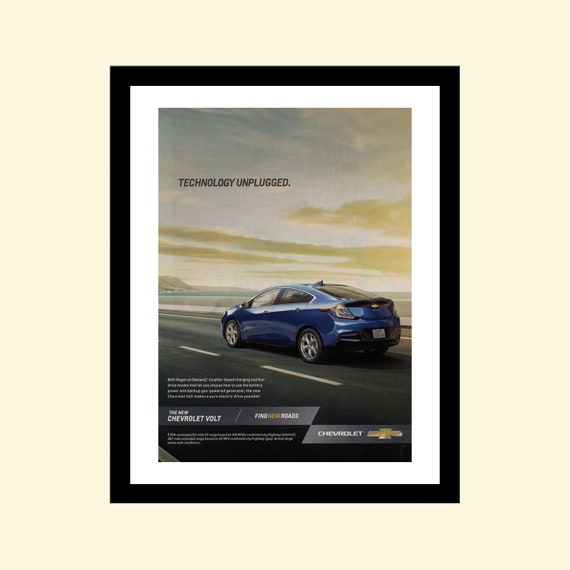The square-shaped image, measuring approximately four inches on each side, presents a detailed advertisement for the Chevrolet Volt. The background is a soft, light yellowish cream, complementing a prominent central rectangle that is around two inches high by an inch and a half wide. This central rectangle is bordered first by a thin black frame, then by a slightly thicker white frame, giving it a polished and contained appearance.

Inside the framed area, a four-door blue Chevrolet Volt sedan, characterized by its intricate aerodynamic design and black wheels, is depicted driving diagonally from the right to the upper left on a two-lane road marked with white dashed lines. The road, rendered in black asphalt, contrasts with the bluish-gray sky above, which features brownish clouds.

In the upper left corner, the advertisement prominently displays the phrase "Technology Unplugged" in black print. Below the vibrant image of the car, there is a paragraph with four lines of white text, though the text is too small to read clearly. Directly beneath this paragraph, the ad announces "The New Chevrolet Volt" and includes the slogan "Find New Roads," with "New" highlighted in a challenging-to-read gold tone. In the lower right-hand corner, the Chevrolet logo and the brand name "Chevrolet" are clearly displayed, concluding the polished and visually engaging promotional piece.